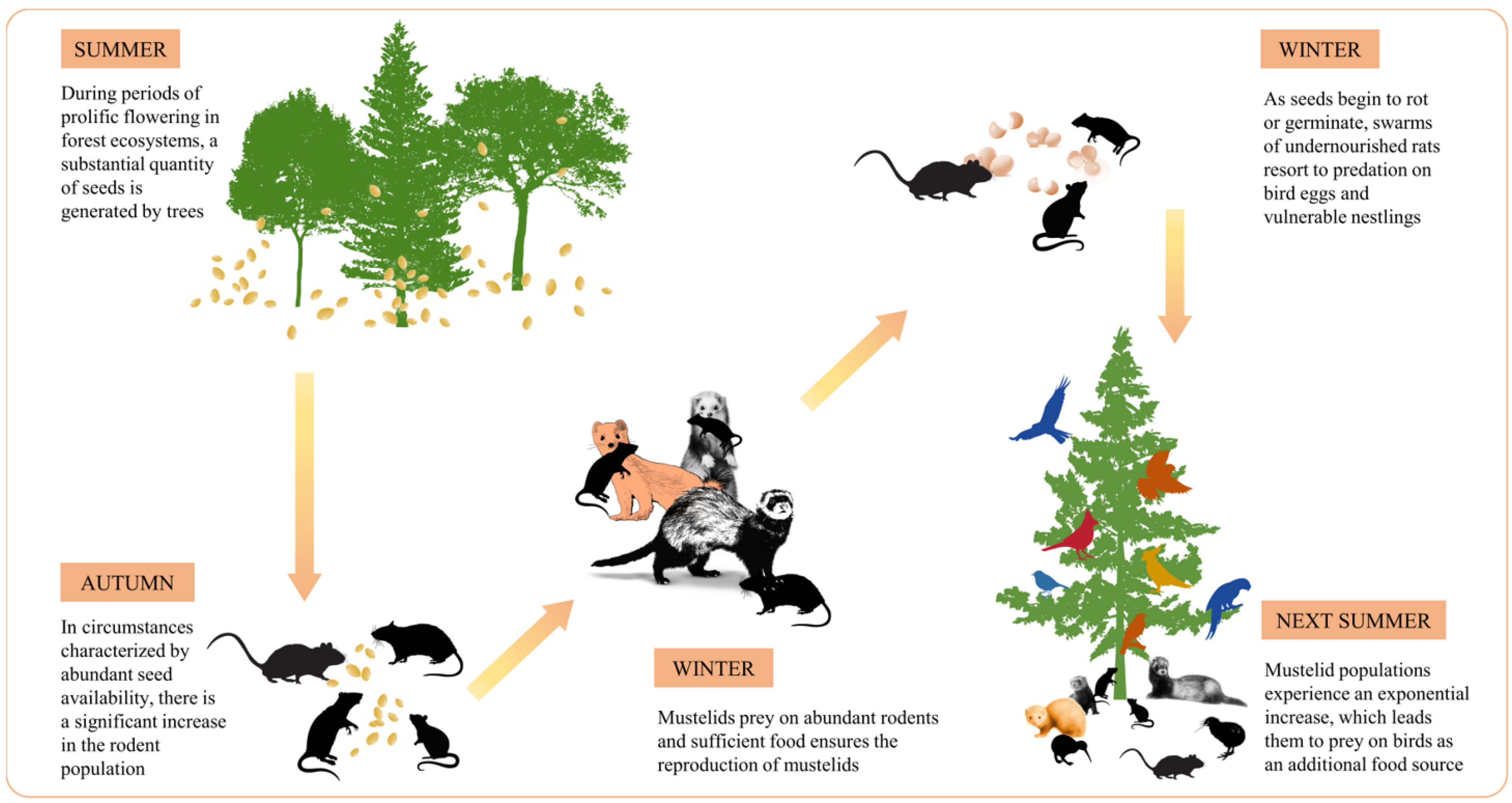The image is a comprehensive illustration depicting the seasonal impact on forest ecosystems through a detailed naturalist explanation. The diagram is organized on a plain white background with five distinct illustrations connected by yellow to red gradient arrows, indicating the flow of events across different seasons: top left to bottom left, bottom left to center, center to top right, and top right to bottom right. Each section is accompanied by black text on an orangey-brown background explaining the seasonal events.

In the top left corner, labeled "Summer," tall green trees are shown, with seeds falling, indicating prolific seed production. The descriptive text highlights that during periods of prolific flowering, trees generate substantial quantities of seeds.

An arrow leads to the bottom left corner for "Autumn," where silhouettes of rats and mice are depicted consuming these seeds. The text explains that the abundance of seeds leads to a significant increase in the rodent population.

From here, an arrow points to the central part labeled "Winter," illustrating mustelids like minks, ferrets, and weasels preying on the abundant rodents. The description notes that sufficient food ensures these mustelids' reproduction.

The flow continues with an arrow going to the top right, also marked "Winter." Here, the imagery shows rats scavenging bird eggs and nestlings as seeds begin to rot or germinate, causing undernourished rats to decimate bird populations.

Lastly, an arrow leads to "Next Summer" in the bottom right, showing a tree with diverse birds like cardinals, blue jays, and bluebirds, along with ground-dwelling birds, mice, rats, and mustelid predators underneath. The text describes how the mustelid populations exponentially increase, leading to additional predation on birds.

This detailed diagram underscores the cyclical nature of seasonal changes and their profound effects on tree seed production, rodent population dynamics, and predator-prey relationships within forest ecosystems.